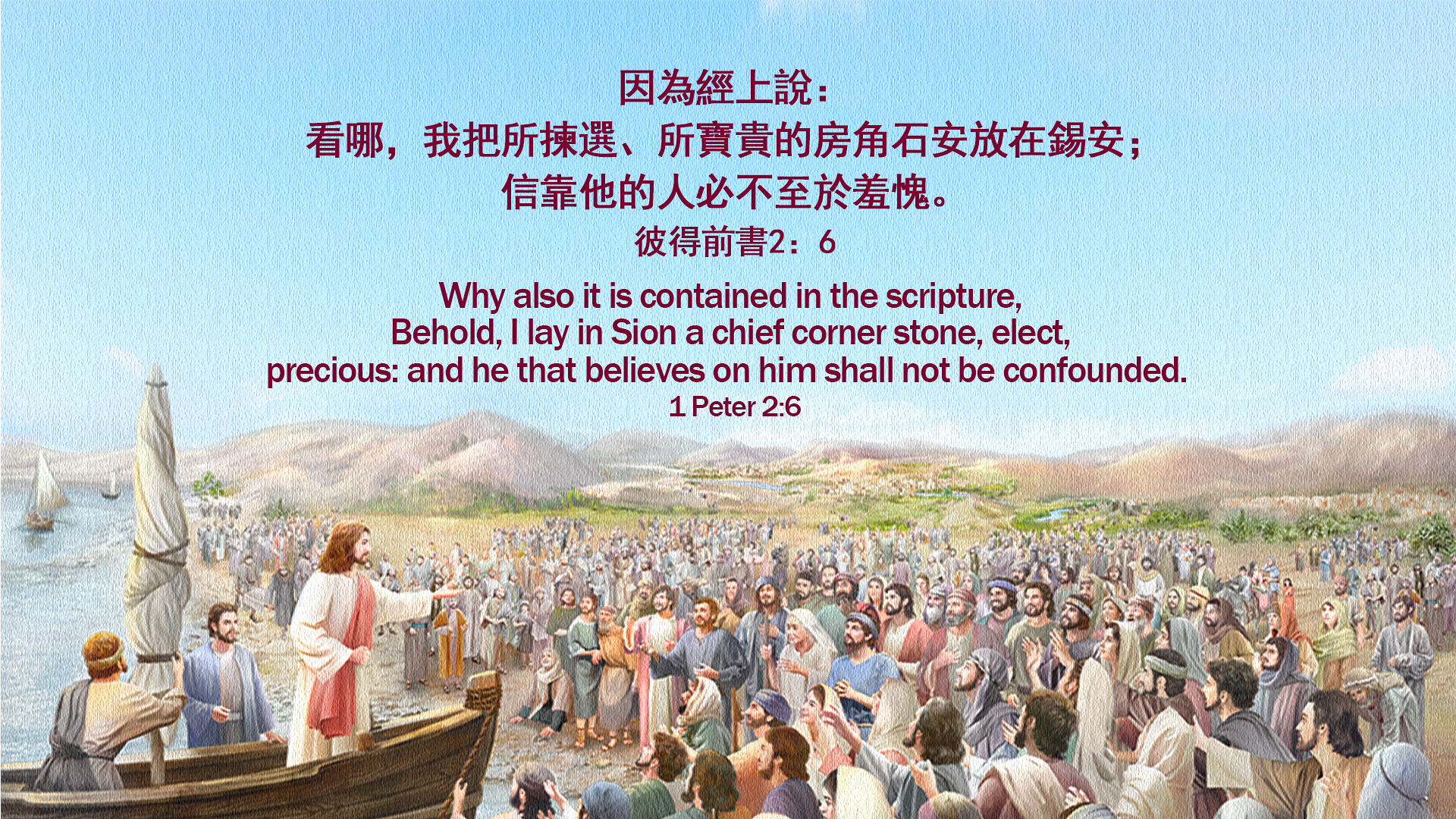This detailed horizontal rectangular image depicts a biblical scene featuring Jesus standing in the prow of a boat with furled sails, addressing a massive crowd on the beach. Jesus, clothed in a light-colored robe, extends his left arm towards the attentive crowd, some of whom are reaching out in return. Behind Jesus, two followers are present—one aboard the vessel and another on the shore.

In the background, gray mountains rise majestically above a verdant landscape dotted with trees and a stream or river winding through it. The sky is a soft blue, adorned with text in an Asian language above a Biblical quote in brown letters from 1 Peter 2:6: "Behold, I lay in Zion a chief cornerstone, elect, precious, and he that believes on him shall not be confounded." The scene captures a moment of profound spiritual connection, with hundreds, if not thousands, of people gathered to hear Jesus speak.